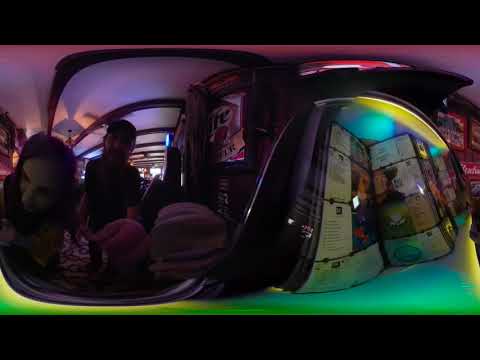In this image, taken with what appears to be a stereoscopic lens, we see a close-up shot focusing on two young, shadowy figures on the left, possibly a man and a woman, both Caucasian and likely under 30. The man, identifiable by his cap and facial hair, extends his finger toward the camera, suggesting the photo was captured from a machine. The setting is an indoor area with a dimly lit atmosphere, enhanced by striking purple, pink, red, and fluorescent green lights, reminiscent of a bar, nightclub, or concert venue. To the right, a neon green arcade-like machine, which resembles a jukebox adorned with posters and CD artwork, adds to the vibrant yet slightly grungy ambiance. The surrounding details, including a light-colored ceiling and scattered projections, contribute to an overall impression of a lively, perhaps slightly divey, nightlife event.